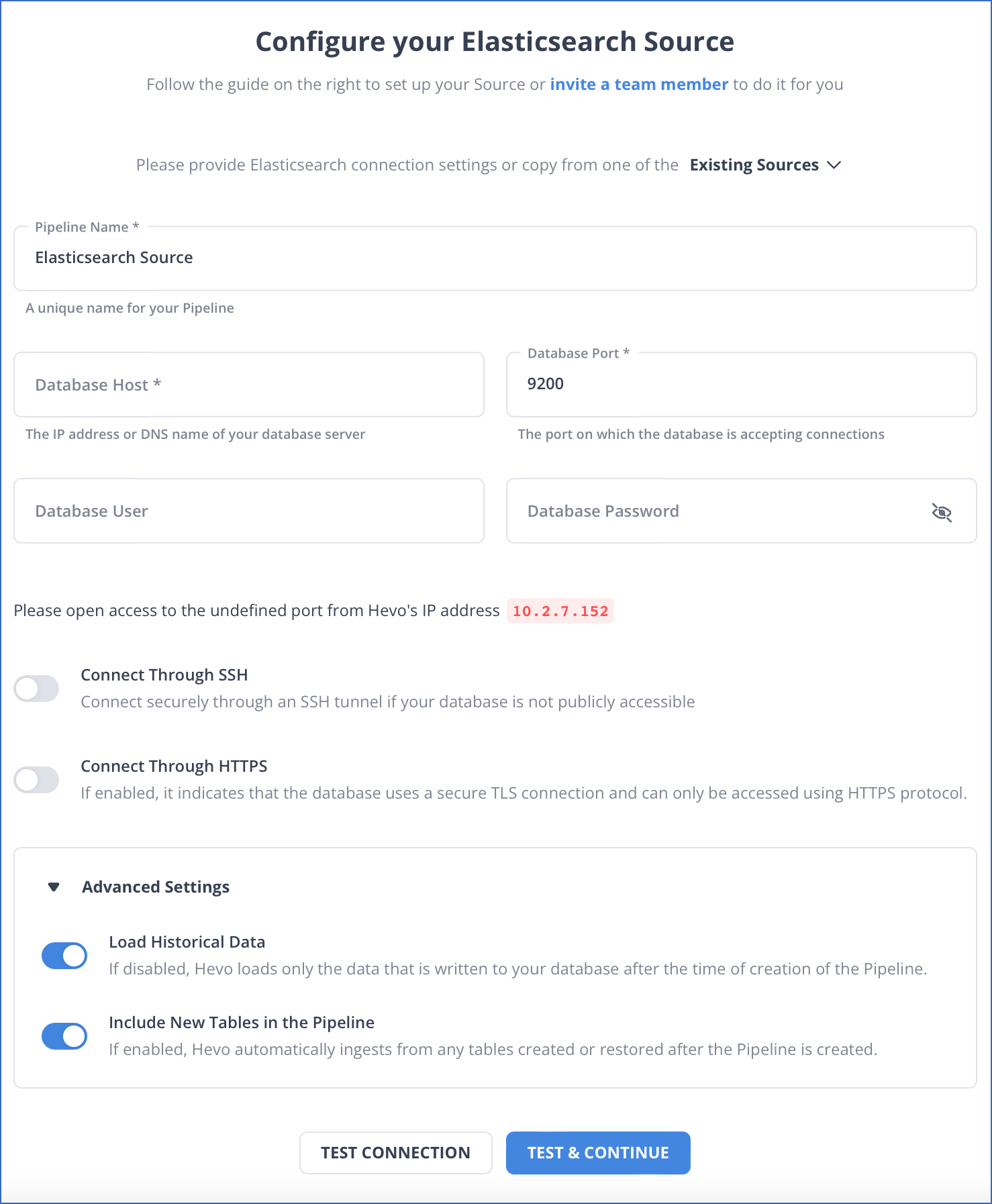In this instructional image for configuring your Elasticsearch source, detailed guidance is provided on the right side to help users set up their source or invite a team member to complete the setup. Users are instructed to provide Elasticsearch connection settings or duplicate one from an existing source.

Key fields and their descriptions include:
- **Pipeline Name:** A unique name for your data pipeline.
- **Elasticsearch Source:** Reference to the source, requiring specification of the database host and port.
- **Database Host:** The IP address or DNS name of your database server, indicated with an asterisk to denote a mandatory field.
- **Database Port:** Defaulted to 9200.
- **Database User and Password:** Credentials necessary for accessing the database.
- **Open Access:** Users are prompted to ensure access to the specified port (undefined) from the specified IP address 10.2.7.152, referred to here as HAGO's IP address.
- **Connect through SSH:** An option to securely connect via an SSH tunnel if the database isn't publicly accessible, noted with a toggle switch currently in the "off" position.
- **Connect through HTTPS:** An additional connection setting that, when enabled, indicates secure TLS connections are required, accessible only via HTTP protocols.

Overall, the image serves as a comprehensive setup guide for configuring an Elasticsearch source with necessary database details and security settings.